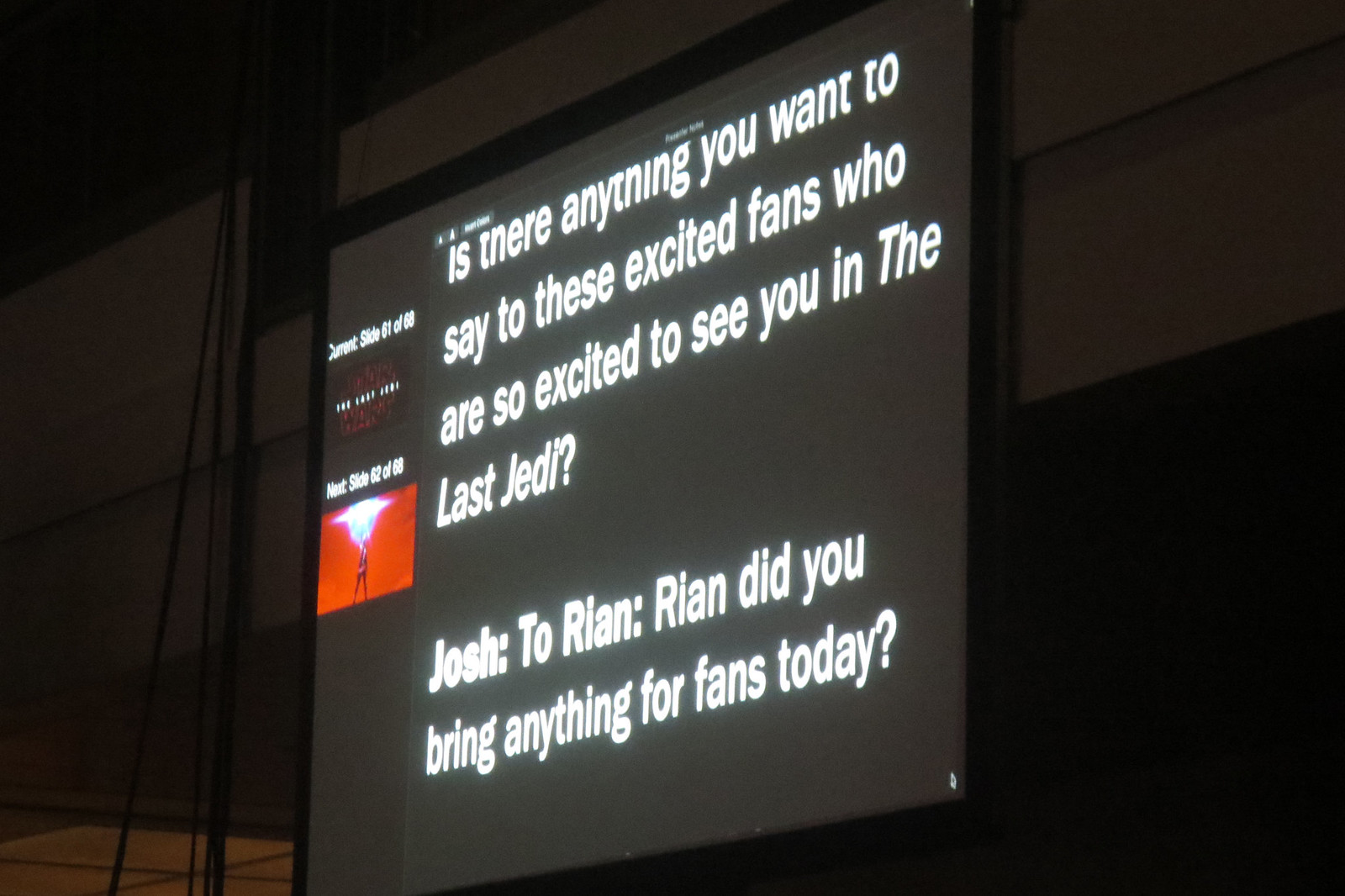This is a nighttime photograph taken outdoors, depicting a large, tilted jumbotron screen attached to a structure, possibly a stadium or indoor coliseum. The image is dark, with the upper left and lower right corners in plain black. The screen itself has a black background with white text that reads: "Is there anything you want to say to these excited fans who are so excited to see you in The Last Jedi?" Below this, it continues with "Josh to Rian: Rian, did you bring anything for fans today?" To the left of this text, there is an orange logo or red stamp. Additionally, the screen displays a slide counter indicating it is "Current slide, 61 of 68" and "Next slide, 62 of 68." The background around the screen appears white, almost like molding, and the bottom of the photo shows a glimpse of a wooden floor with metal poles extending upwards.